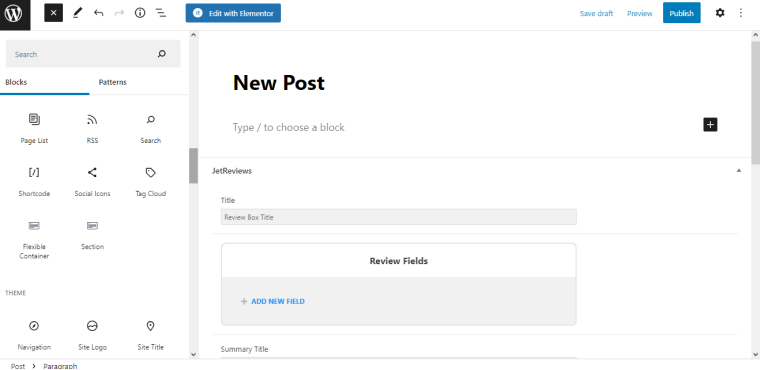**Caption:**

The image displays the interface of a WordPress website, specifically the screen for creating a new post. The top of the page prominently features a "New Post" heading. On the left sidebar, a distinctive 'W' logo within a white circle on a black background, indicative of WordPress, is visible. Below this logo, a black box with a white 'X' inside serves as a close option. Additionally, common interface icons such as an edit icon, 'go back' and 'go forward' arrows, an information 'i' in a circle, a menu represented by three stacked lines, and a magnifying glass icon for search functions are displayed.

The main section is divided into two tabs: "Blocks" and "Patterns," with the "Blocks" tab highlighted in blue, signifying its active state. Within the "Blocks" section, various options are listed, such as Page List, RSS Search, Shortcode, Social Icons, Tag Cloud, Flexible Container, and Sections. Under a subsection titled "Theme," options include Navigation, Site Logo, Site Title, and, once more, Navigation. 

On the right side, "Post" is shown followed by a right arrow and options for Paragraph and 'Edit with Elementor.' Below these, an interface prompt states "New Post," inviting users to "Type to choose a block." Additional options for integrating Jet Reviews, including Title, Review Box Title, and Review Fields, are also displayed. A blue button labeled "Add New Field" with a plus sign concludes the setup, inviting further customization of the review fields.